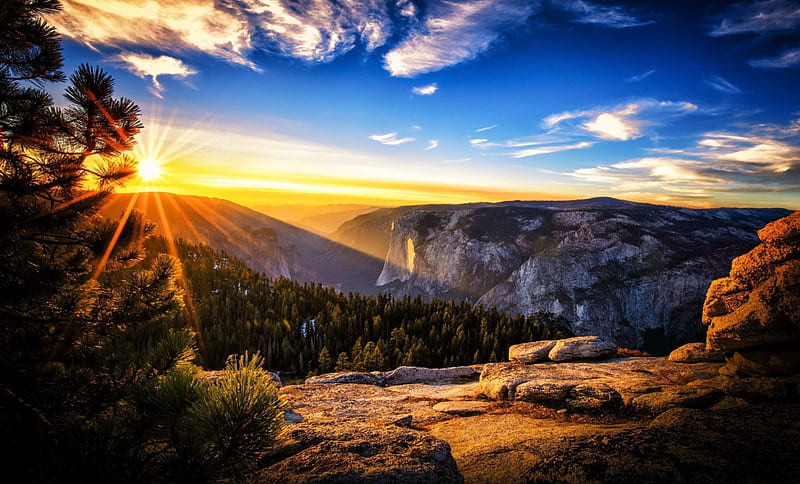This captivating image showcases a breathtaking mountain vista, bathed in the gentle light of either sunrise or sunset. In the foreground, an uneven arrangement of brown and gray stones forms a natural viewing platform, inviting one to stand and soak in the awe-inspiring scenery. A vibrant green bush and a resilient pine tree lend fresh life to the rugged terrain. Beyond, a lush pine forest stretches across rolling hills, creating a verdant sea of green. Farther in the distance, a series of grand mountains rise majestically, their peaks shrouded in a serene, dreamlike atmosphere. The sky above is a mesmerizing blend of yellow, white, and blue hues, painted in dynamic strokes as if captured in mid-motion. Wisps of clouds appear to glide across the expanse, softening the scene with their ethereal presence. This moment, frozen in time, perfectly encapsulates the tranquil splendor of a mountain landscape embraced by the dawning or waning light.